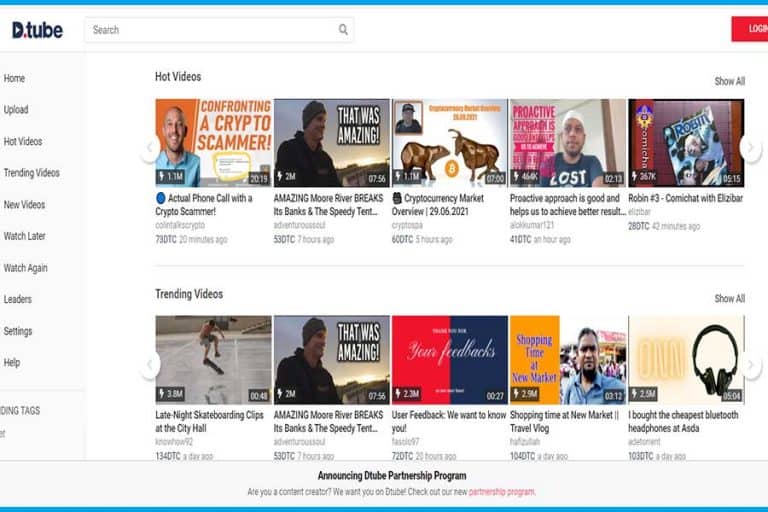DTUBE Homepage Overview:

The DTUBE homepage features a minimalist design with a predominant white background. At the center, there's a prominent search box for easy navigation.

On the left side, a vertical menu lists navigation options:
- Home
- Upload
- Hot Videos
- Trending Videos
- New Videos
- Watch Again
- Leaders
- Settings
- Help
- Tags

Highlighted 'Hot Videos':
1. **Confronting a Crypto Scammer**: This video showcases a compelling phone call confrontation with a crypto scammer.
2. **Getting More River Breaks Its Banks and the Speedy Tent**: Features a man standing by a flooding riverbank.
3. **Cryptocurrency Market Overview**: An informative video featuring a bear and a moose.
4. **Proactive Approach is Good and Helps Us to Achieve Better Results**: A man wearing a do-rag and a T-shirt with "Lost" discussing the benefits of a proactive approach.
5. **Robin 3, Come and Chat with Elizabeth**: An invitation to engage in conversation with Elizabeth.
6. **Late Night Skateboarding Clips at the City Hall**: Highlights thrilling skateboarding footage filmed at City Hall.
7. **User Feedback: We Want to Know You**: A video calling for user feedback.
8. **Shopping Time at New Market**: A shopping adventure at a new market.
9. **Travel Vogue**: A travel-themed video.
10. **I Bought the Cheapest Bluetooth Headphones at Asda**: A review of budget Bluetooth headphones from Asda.

An announcement at the bottom addresses content creators:
"Announcing DTUBE Partnership Program: Are You a Content Creator? We Want You on DTUBE. Check Out Our New Program."